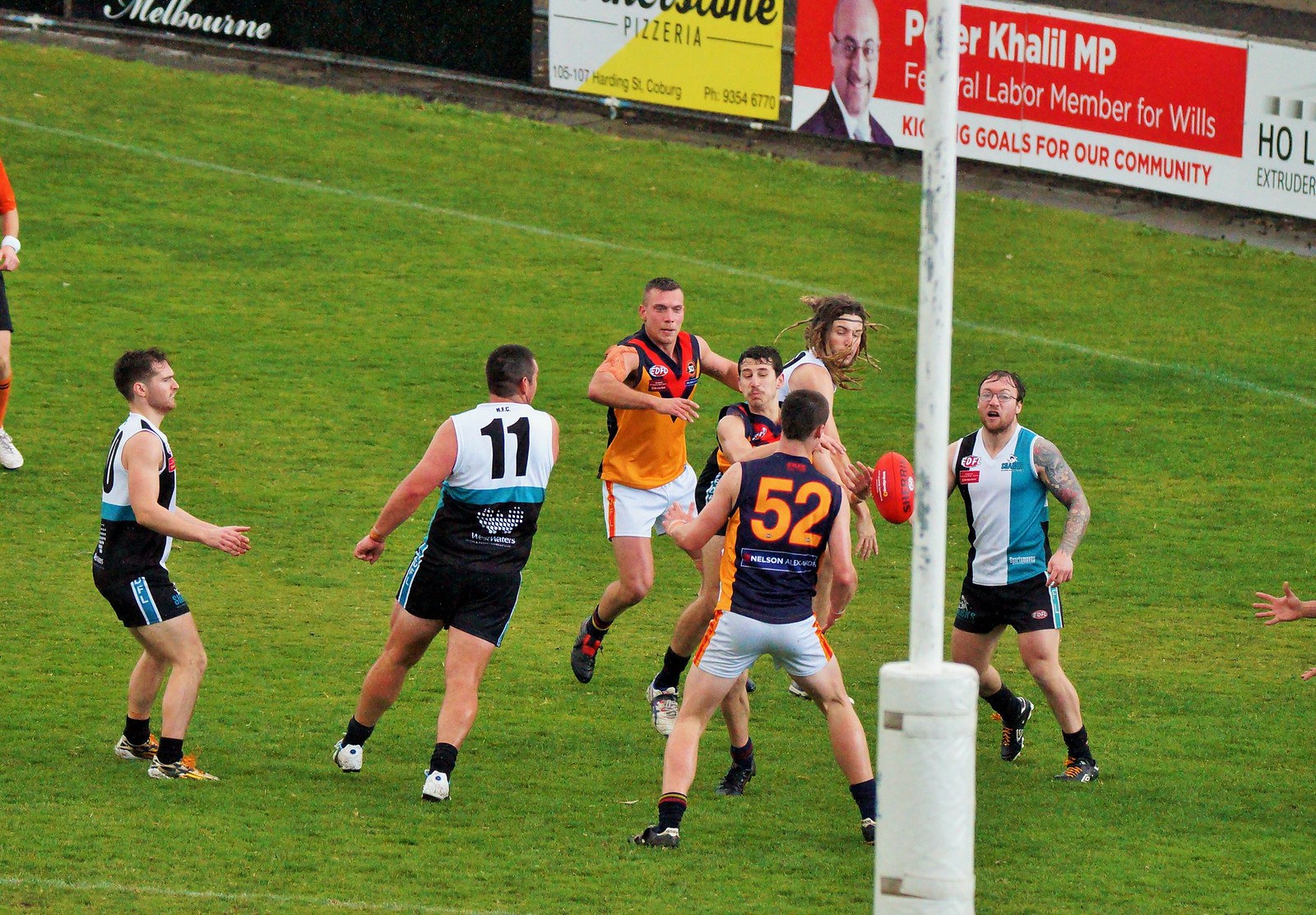In this detailed image of a rugby match taking place on a vividly green grass field within an arena decorated with posters along its perimeter, nine players are visible, divided into two teams. The teams are distinguished by their uniforms; one set of players is wearing blue, white, light blue, and black jerseys with black shorts, while the other set is clad in black, gold, and white jerseys with matching shorts. The scene shows the players congregated in a compact area towards the center of the image, focusing on a central figure with black hair who appears to be exerting force against an opponent immediately in front of him. This central player, near the 52-yard line, holds an orange football in his right hand. Nearby, another player is slightly backed off to the left, possibly preparing to catch the ball. Two other players are partially visible: one at the top left edge of the image, showing only part of his arm and leg, and another at the bottom right with only his hands in view. Additionally, a white pillar with a cylindrical base is seen in the center-right part of the image.